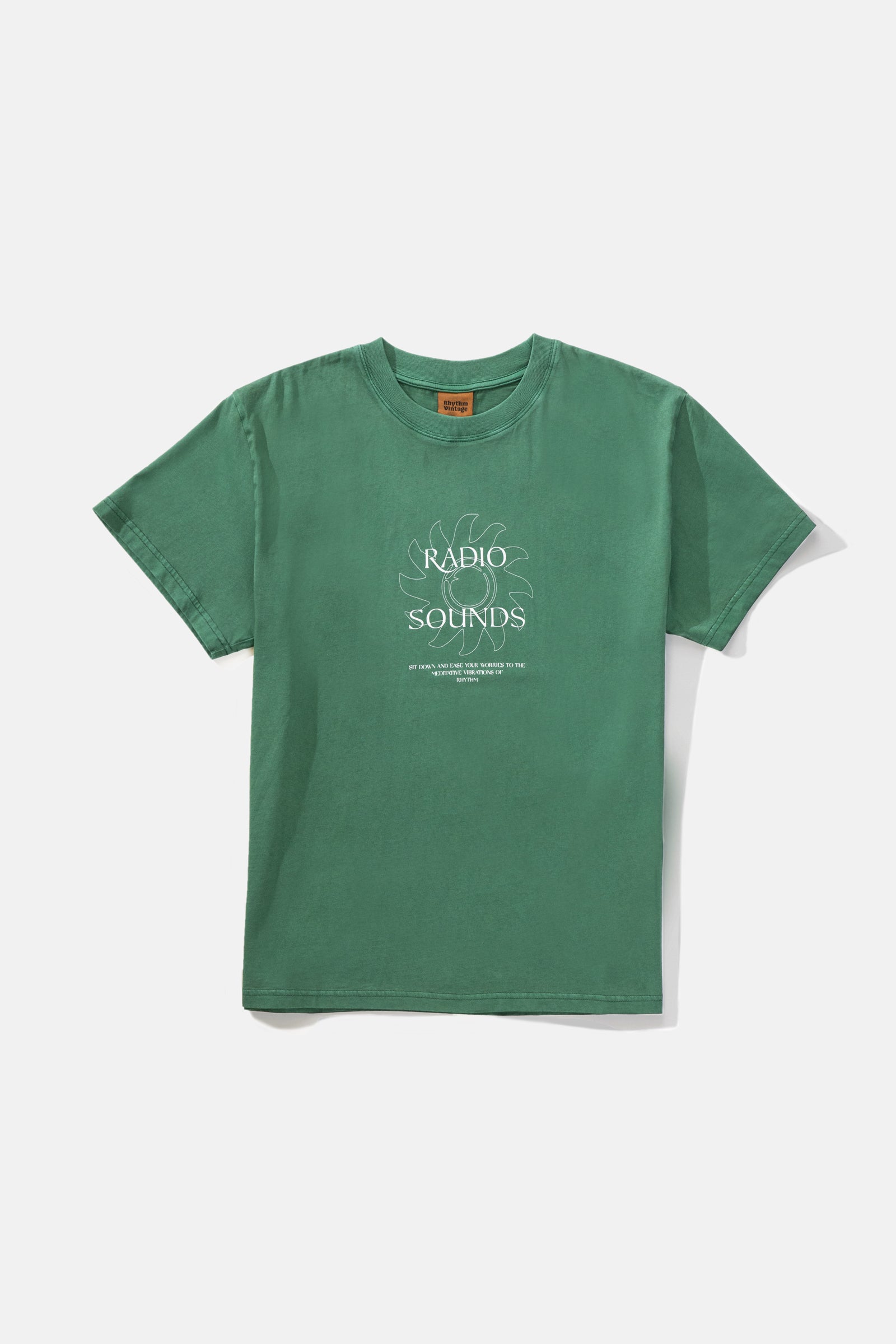The image depicts a professionally photographed green t-shirt set against a light gray or off-white background. The short-sleeve shirt, appearing to be made of a heavier cotton material, features a brown tag at the collar, imprinted with indistinct black writing. In the center of the t-shirt is a white outlined design resembling a sun or pinwheel, with "Radio Sounds" written in white font above it. Beneath the sun icon is additional text that is too small to discern. The shirt also casts a subtle gray shadow, enhancing the professional quality of the photograph likely intended for advertising purposes.